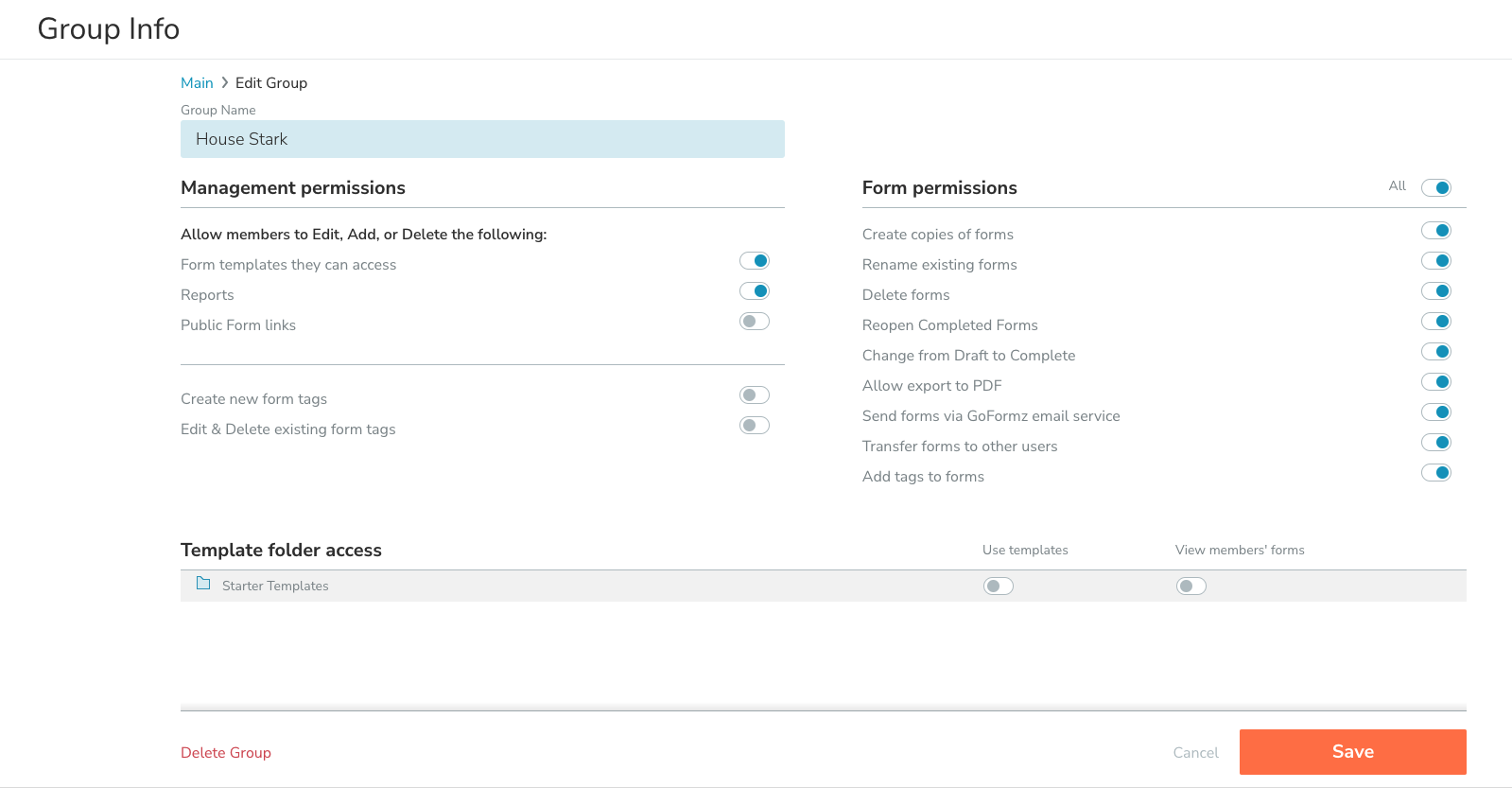This image portrays a simple webpage interface designed for group management. The entire background is white, and the content is structured in a clean, straightforward manner. 

At the top-left corner, the heading "Group Info" is displayed in black letters. Directly below it, there's a navigational breadcrumb that reads "main / edit group," indicating that users can return to the main page by clicking "main."

Below the breadcrumb lies a section labeled "Group Name." Within this section, in a light blue input box, the name "House Stark" is typed in black letters.

Following the group name section is the "Management Permissions" area. This area is further divided with a subheading in black ink stating, "Allow members to edit, add, or delete the following." Under this heading are three toggle options:

1. **Form Templates they can access**: This toggle is turned on, indicated by the teal dot positioned to the right.
2. **Reports**: This option is also enabled, as shown by the similar teal dot.
3. **Public Form Links**: This toggle is turned off, visible from the grayed-out button and dot.

A horizontal line demarcates the next subsection, which lists two additional permissions, both turned off:

1. **Create New Form Tags**
2. **Edit and Delete Existing Form Tags**

To the right side of the image, there is a section titled "Form Permissions." This area contains nine different selections, all of which are toggled on. These selections include options like "Create Copies of Forms," "Allow Export to PDF," and "Add Tags to Forms."

Further down, though not at the very bottom, there is a subsection labeled "Template Folder Access" with additional choices for managing access to template folders.

Finally, at the bottom of the interface, there are two red words: "Delete Group," indicating an option to remove the group. Adjacent to this are two action buttons: a prominent "Save" button on the far right and a "Cancel" button, providing options to either save the settings or cancel the changes made.